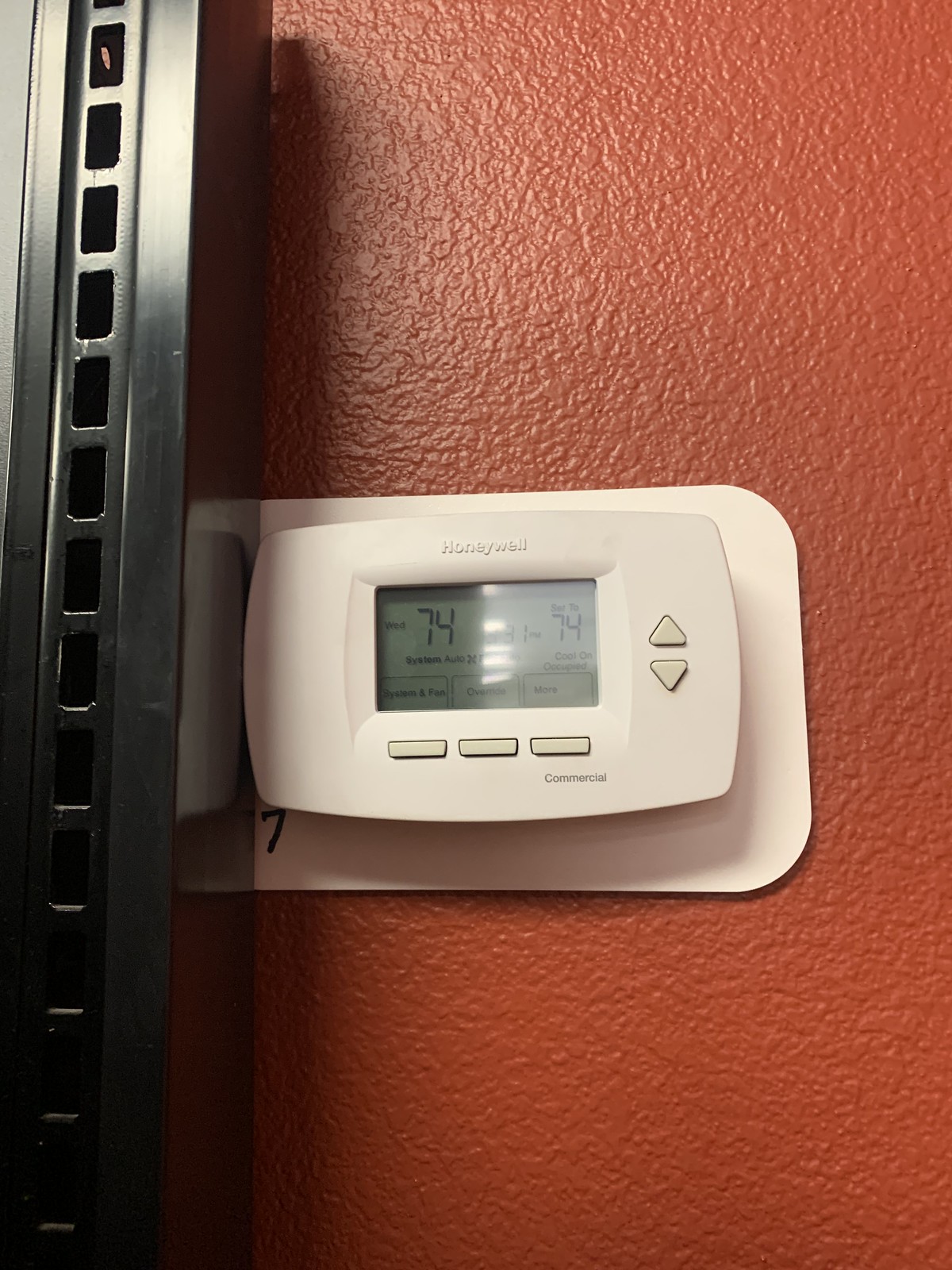This photograph captures a textured and visually distinct wall painted in a rough, reddish, brick-like color, reminiscent of sandpaper due to its uneven surface and prominent horizontal and vertical lines. On the left side of the image, a stark black bar runs vertically from the bottom to the top edge, featuring a series of vertical rectangular cut-outs arranged in a straight line down its center. Affixed to this black bar, near its midpoint, is a temperature thermostat for an air conditioning unit. The thermostat is mounted on a white, rounded rectangular plate and encased in a clear plastic cover. The device, branded Honeywell at the top, includes a digital display reading 74 degrees. Below the screen are three rectangular buttons, with two arrows—one pointing up and the other down—indicating temperature adjustment controls.